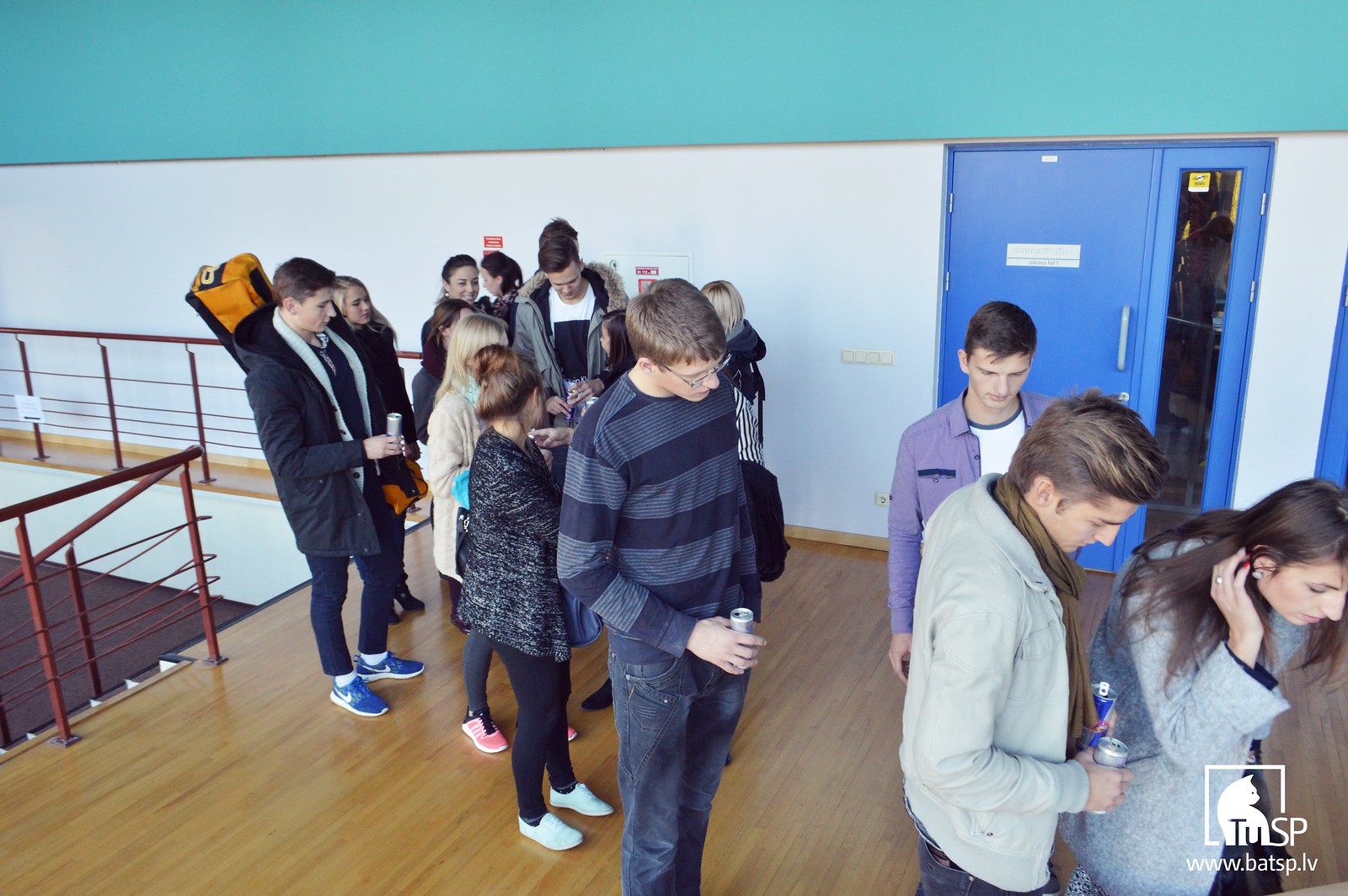The image depicts a group of approximately a dozen mixed-gender individuals, presumably school-aged, waiting in line within an indoor setting. The queue stretches from the left to the right and includes people holding energy drinks, notably Red Bull. The flooring beneath them is brown hardwood, and they are positioned next to a staircase with a prominent red metal railing on the left side. Behind them, a white wall features a blue door with a turquoise upper section. In the bottom right corner, a watermark shows a square logo with a transparent interior containing a white cat and the text "TUSP" beneath it. Accompanying this logo is the URL "www.bats.lv" in white lettering. The setting gives the impression of being on the top floor of a building, possibly a gym area, considering the arrangement of railings and steps.